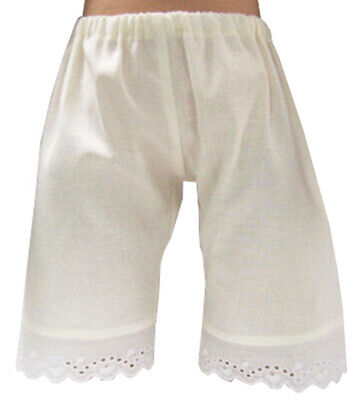This photograph showcases a pair of women's white bloomers, likely made from a cotton or linen material, set against a white or slightly transparent background. The bloomers feature an elasticated waistband which appears slightly bunched, indicating a drawstring or ruched design. The bottom of the bloomers extends just below the knees and is adorned with a delicate scalloped lace trim, often described as having a borderet anglaise effect. The fabric is lightweight and somewhat sheer, revealing a hint of the underlying material. The bloomers exhibit a faint stripe just above the lace trim, adding a subtle decorative element. The image suggests a studio setting, illuminated by a soft, possibly yellowish artificial light. The mannequin torso, possibly a dummy, wearing the bloomers shows a small portion of skin tone at the top, emphasizing the slightly transparent nature of the fabric. The overall look is both delicate and vintage, reminiscent of classic female undergarments.